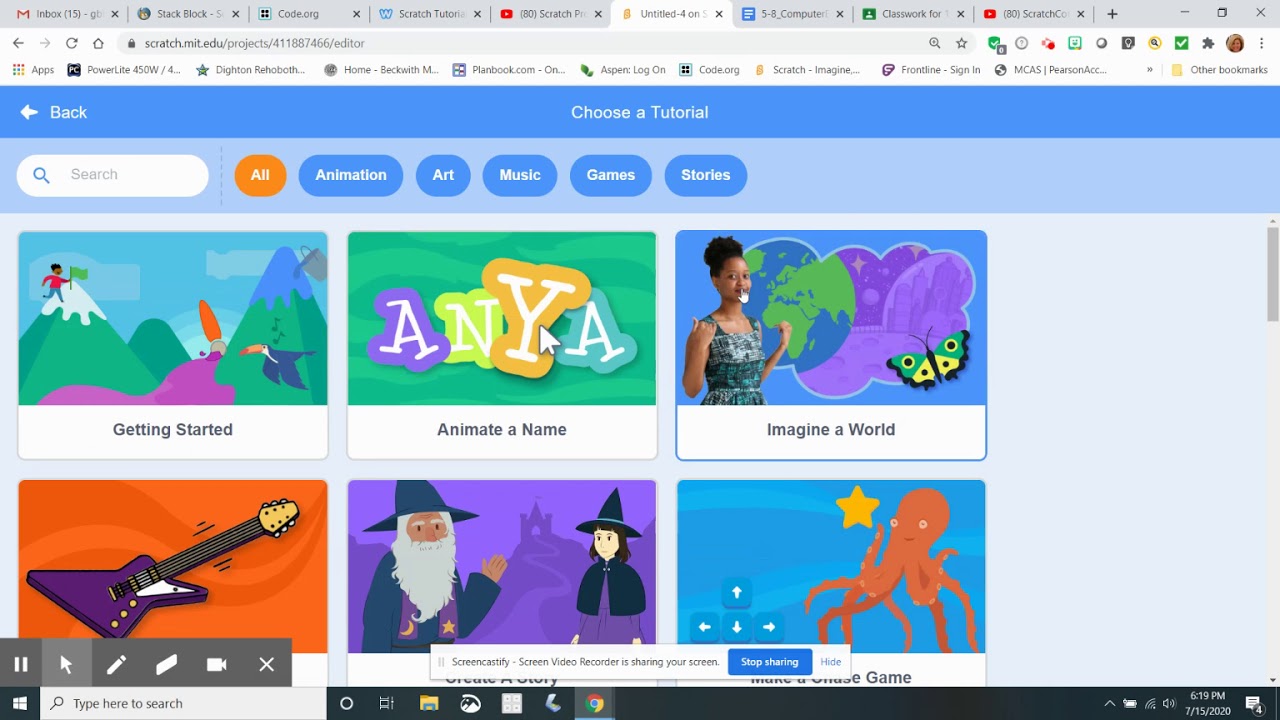This image is a screenshot of a vibrant and colorful website, designed with a children's audience in mind, featuring numerous cartoony elements. The screenshot captures a browser window, showing the user has nine open tabs. These tabs include two YouTube tabs (both seemingly related to "Scratch"), Gmail, something called Stackblock, Code.org, a Scratch tutorial, a Google Docs document, and an Excel sheet labeled as classwork.

The primary webpage displayed in the screenshot is a tutorial page on Scratch, indicated by the URL "scratch.mit.edu" and the header text "Choose a tutorial." The website features a navigation bar with categories such as All, Animation, Art, Music, Games, and Stories. The "All" category is currently highlighted in orange, suggesting it is the active section. Below the navigation bar, various games or page options related to the selected category are visible, hinting at the extensive variety of content available for users to explore.